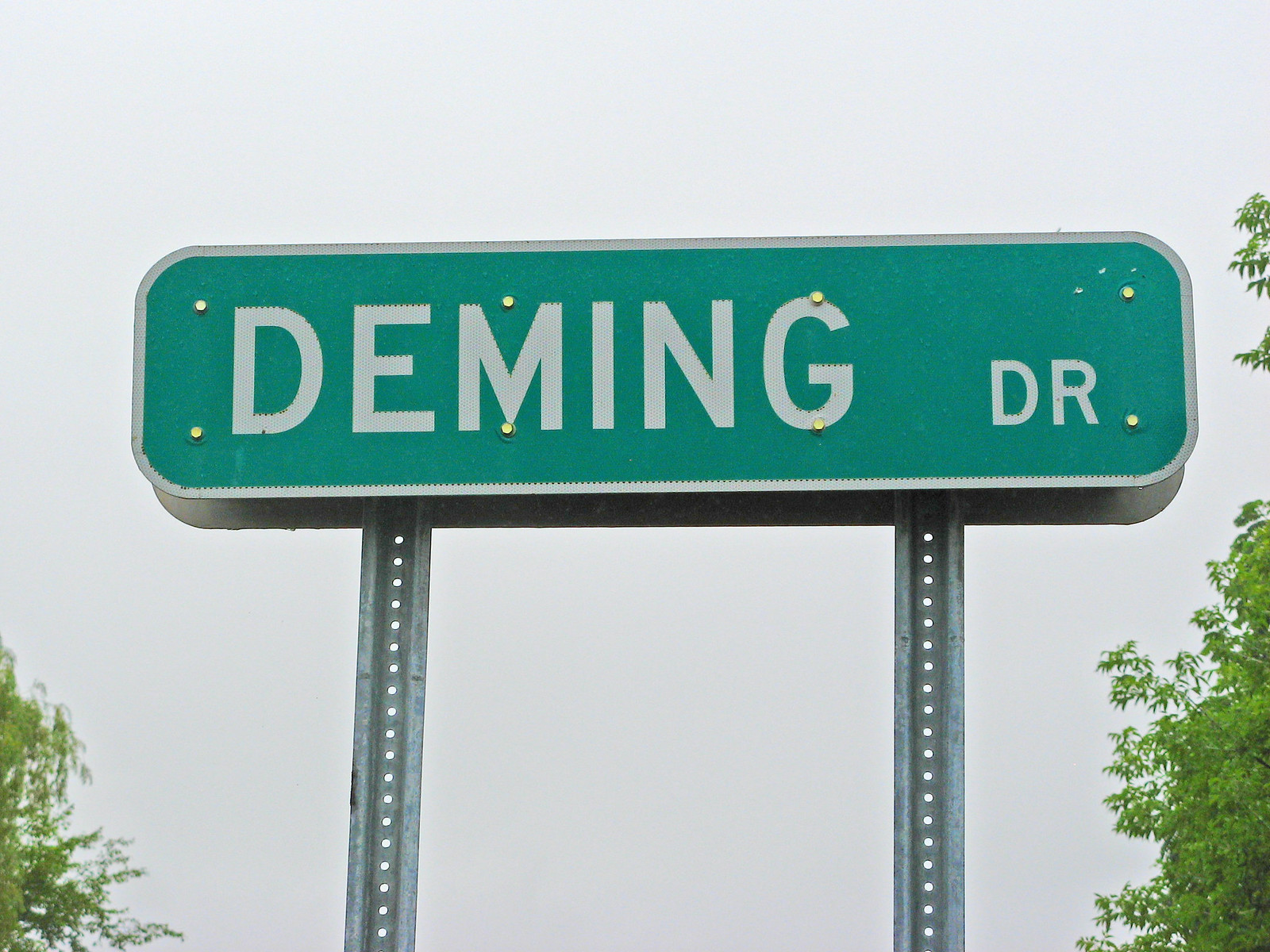This image features a green street sign with white lettering displaying "Deming Drive." It is mounted on two silver poles, each characterized by a series of small, hollow dots running vertically. The poles anchor the sign to the ground. The rectangular sign has rounded edges and showcases several small yellow circles across its surface, with some centered and others positioned toward the edges, totaling eight marks. The background is predominantly gray, suggesting an overcast sky. In the bottom left corner and to the right side of the image, lush green leaves are visible, hinting at nearby trees or bushes. There is also some visible rust on the sign. The overall scene is set against a subdued, grayish backdrop, emphasizing the starkness and simplicity of the street sign and its surroundings.